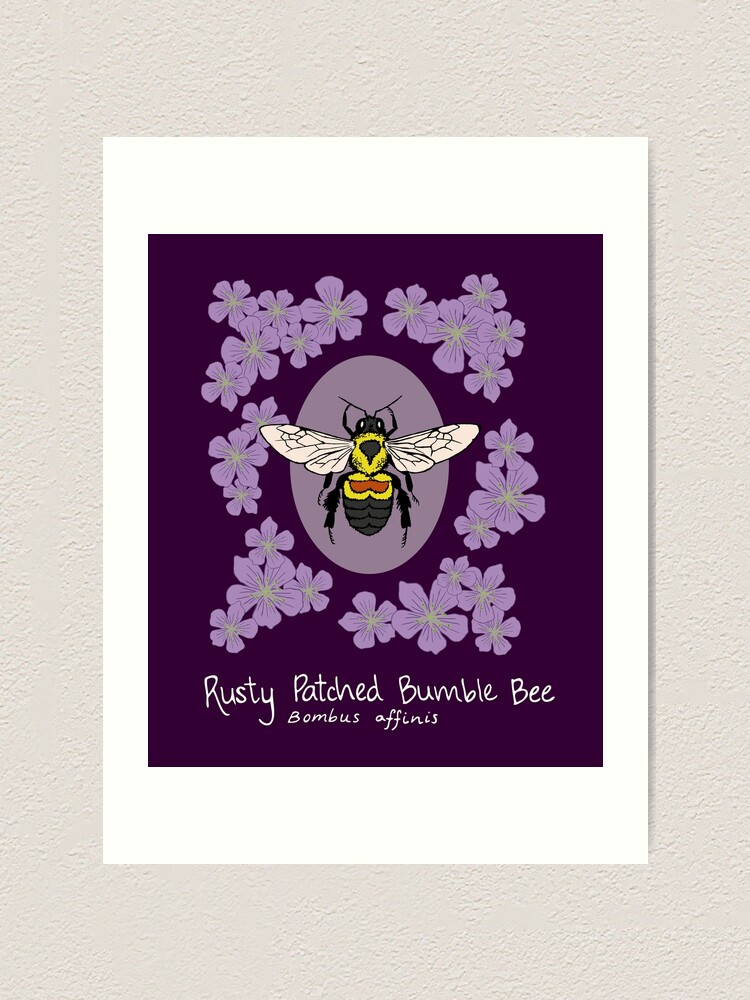The image showcases an artistic poster displayed on a cream-colored, textured stucco wall. The poster, set against a slightly irregular, white-bordered frame, features a predominant dark violet to dark pink background. At the heart of the poster lies an illustrated oval of a similar purple hue. Within this oval is a detailed illustration of a bee, characterized by its yellow body, a prominent red stripe surrounded by yellow, and white wings. Encircling the bee are numerous vibrant purple flowers, each flower consisting of five petals with green centers. Below the central illustration, in white print, the text reads: "Rusty Patched Bumblebee," followed by its Latin name, "Bombus affinis."